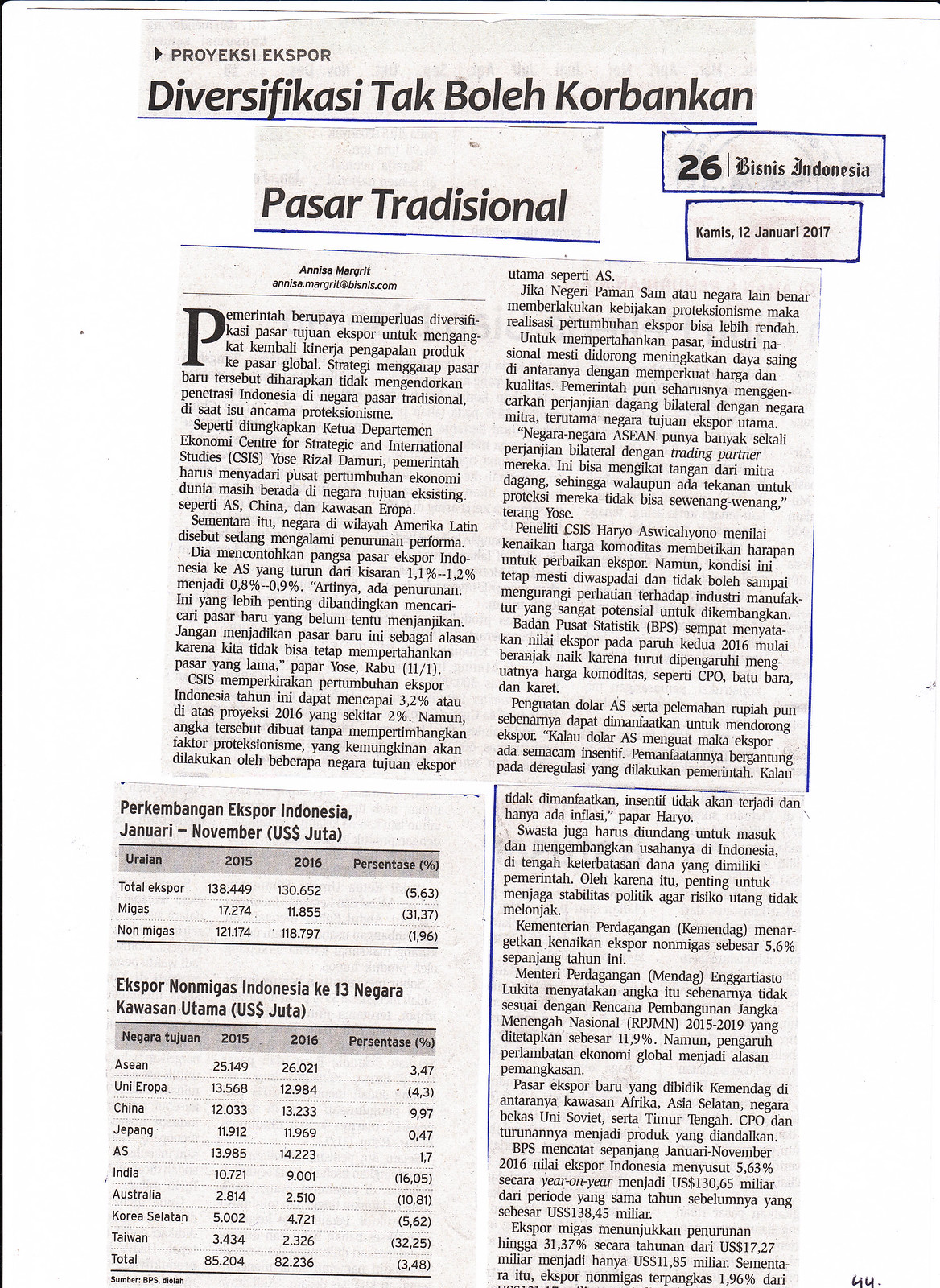The image depicts a scanned newspaper article, primarily in Indonesian, that appears to be a compilation of various clippings pasted onto a white background. The article is slightly tilted to the right, showcasing a mix of off-white and pinkish hues in the newspaper material. At the top, there is a headline with a thin blue line underneath, followed by a sub-headline and the author’s name, Anissa Margrit, along with an email address, suggesting it's a relatively recent publication. The date "12 Januari 2017" is clearly visible, using the Indonesian spelling of January. To the right, the header features two rectangles stacked vertically, one with the number "26" in bold print and the other with some stylized Old English cursive text. Below, the main body of the article consists of two columns, with the first column only extending halfway down the page, making room for a detailed grid of numbers and percentages labeled from January to November, accompanied by a US dollar sign. Multiple paragraphs of text complete the layout, interspersed with blue pen markings circling and boxing various sections, indicating particular points of interest.